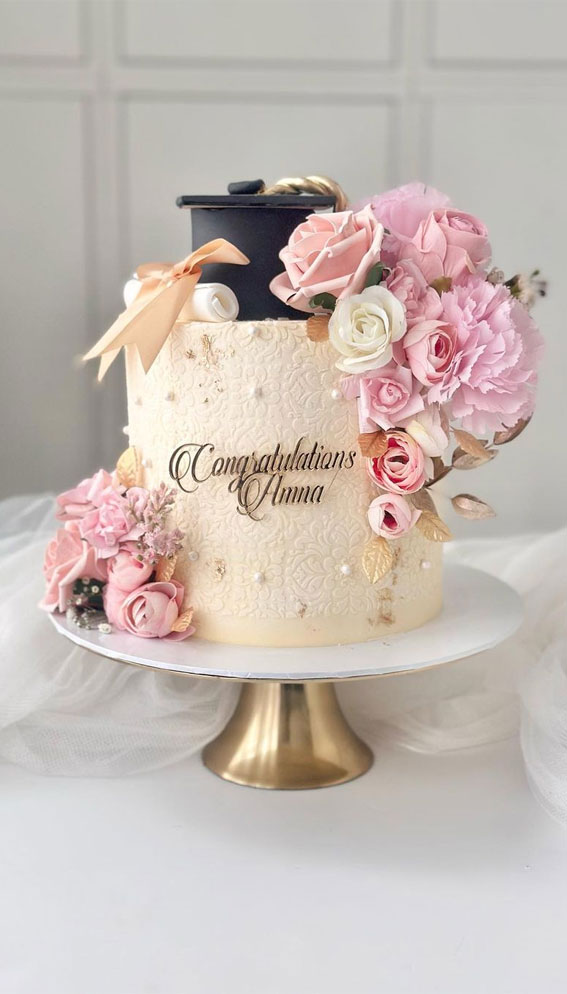The photograph showcases an elegant, tall cylindrical graduation cake, set against a white background with a decorative white wall and white tulle bunched behind it for added beauty. The cake is displayed on a sophisticated gold and white cake stand atop a white table. The cake itself is light beige with delicate pink and white roses adorning the lower left and upper right corners. A black, stylized graduation hat and a fondant diploma with a peach-colored ribbon are artfully placed on top. The front of the cake features the message "Congratulations, Anna" in elegant script, possibly added post-photograph. Edible white and beige beads decorate the cake, complementing the overall fancy aesthetic.